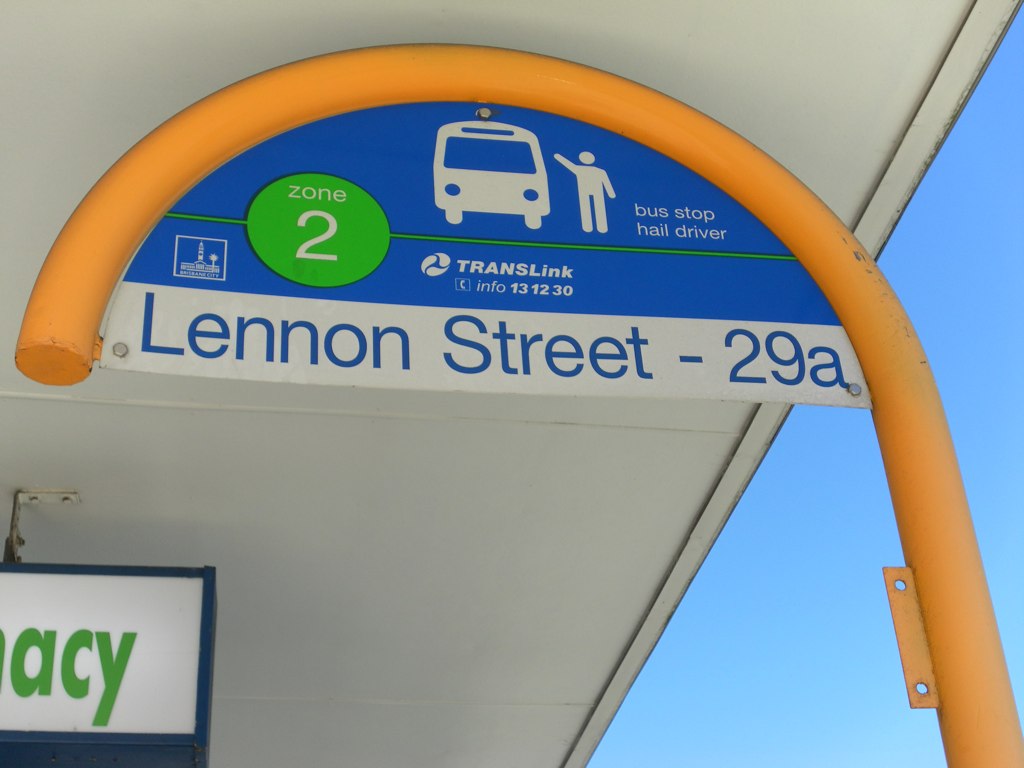This color photograph captures a close-up view of a bus stop sign set against a vibrant blue sky. The sign is mounted on an inverted J-shaped pole, painted in a striking bright yellow. The top portion of the pole supports a beige or gray roof, providing shelter for waiting passengers. The bus stop sign itself is predominantly blue and white, prominently displaying "Lennon Street 29A" in large letters. The sign also features a green circle marked "Zone 2" and an illustration of a bus alongside a stick figure hailing the vehicle, with the words "bus stop hail driver" in white print. Below this illustration, the sign provides additional information: "TransLink Info 131230," accompanied by the TransLink logo. The scene is perfectly framed by the clear, azure sky visible to the right of the sign.